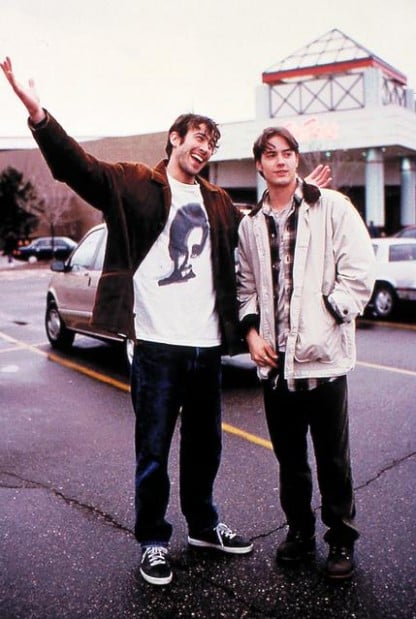This vertically aligned, older photograph captures a daytime scene outside a shopping mall. The sky above is solid light gray, adding to the vintage feel of the image. The background features a store with distinctive white pillars and a red triangular hipped roof awning. In the parking lot, where there are visible cracks in the black speckled concrete and solid yellow lines marking the spaces, several cars, including a silver minivan, are parked.

In the foreground stand two individuals, both with short brown hair that's slightly longer in the front. The person on the left is dressed in dark blue jeans and a white t-shirt featuring a black and white image of a person's head, topped with a brown jacket. Their arms are outstretched, palms up, as they smile broadly at the person next to them. The person on the right is dressed in black pants, a plaid button-down shirt layered over a t-shirt, and a beige jacket. This individual smiles slightly with their arms resting by their sides. It appears the ground is slightly wet, suggesting it may have recently rained, and the overall atmosphere suggests these two friends are enjoying a casual outing together.